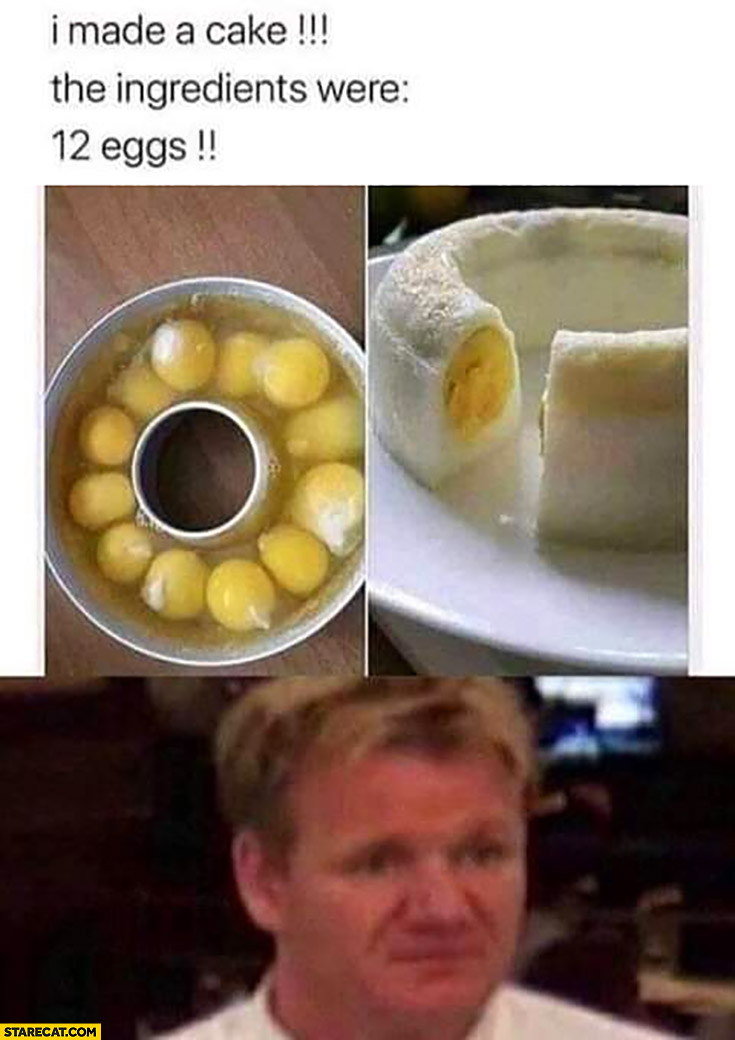In this internet meme, the top half of the image has a white background with three lines of text in a very thin, lowercase black font. The first line enthusiastically states, "I made a cake!!!" followed by, "The ingredients were:" and "12 eggs!!". Below this text, the image is split into two sections. On the left, there is a circular metal cake pan filled with 12 raw eggs on a white-brown wooden table. On the right, a completed angel food cake sits on a white plate, with a noticeable slice cut out. At the very bottom of the image, a smaller, blurred photograph of a neutral-faced Gordon Ramsay in his white chef outfit appears, suggesting his silent judgment. In the bottom left corner, a yellow block watermark reads "staircap.com" in all capitals. The colors predominantly featured are black, white, yellow, and brown.